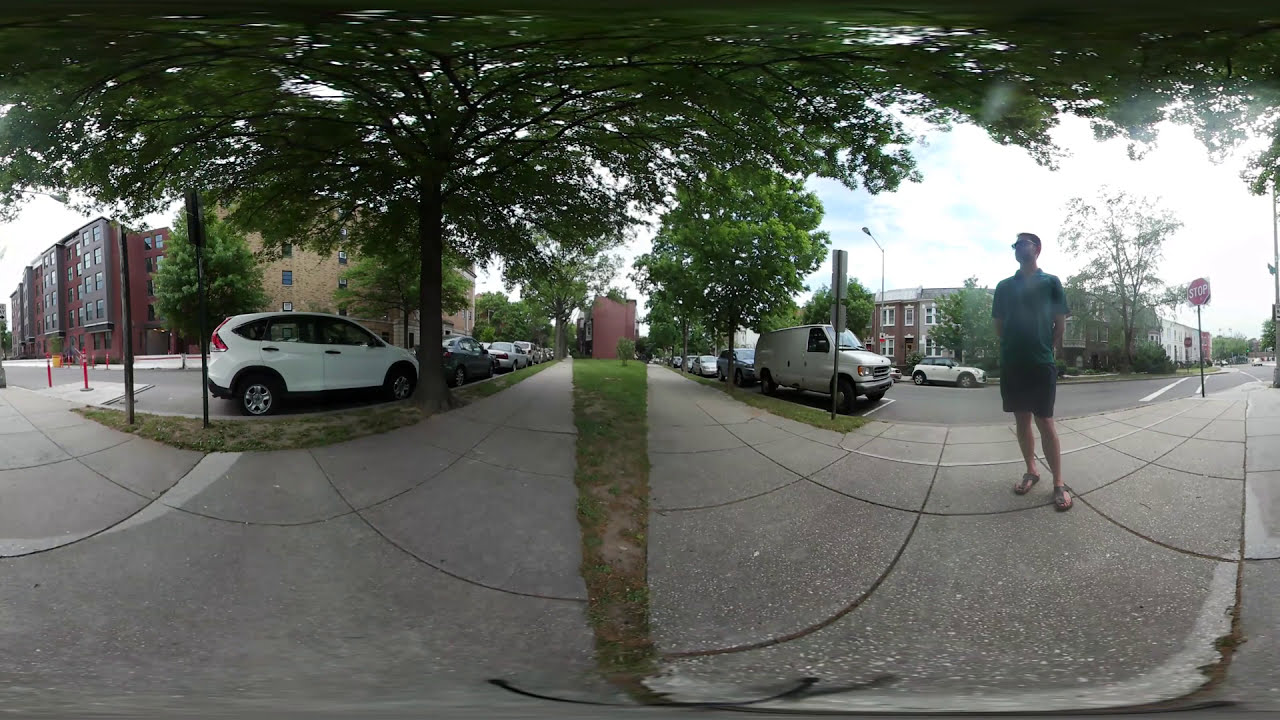This 360-degree image taken on a bright but cloudy day captures a vivid outdoor urban scene. At the center is a small island of green grass and a bit of dirt, dividing two paved walkways. A tall red building rises prominently in the background. The detailed foreground is split into two sides. On the left, there's a large red building with multiple windows, adjacent to a brown brick building. In front of these buildings, several cars are parked beneath a large tree, including an SUV and an older white van without rear windows. The man in the scene stands on a cobblestone sidewalk, wearing a blue polo shirt, black shorts, brown sandals, and sunglasses. He has lighter skin, short black hair, and is looking toward the left. To his right, a red stop sign is also visible. The scene is further accented by patches of green grass, a streetlight, and another set of buildings that appear to be townhomes or attached houses. The roads are paved with gray asphalt, and despite the absence of other people, the image conveys a bright, clear daytime atmosphere with plenty of natural light.